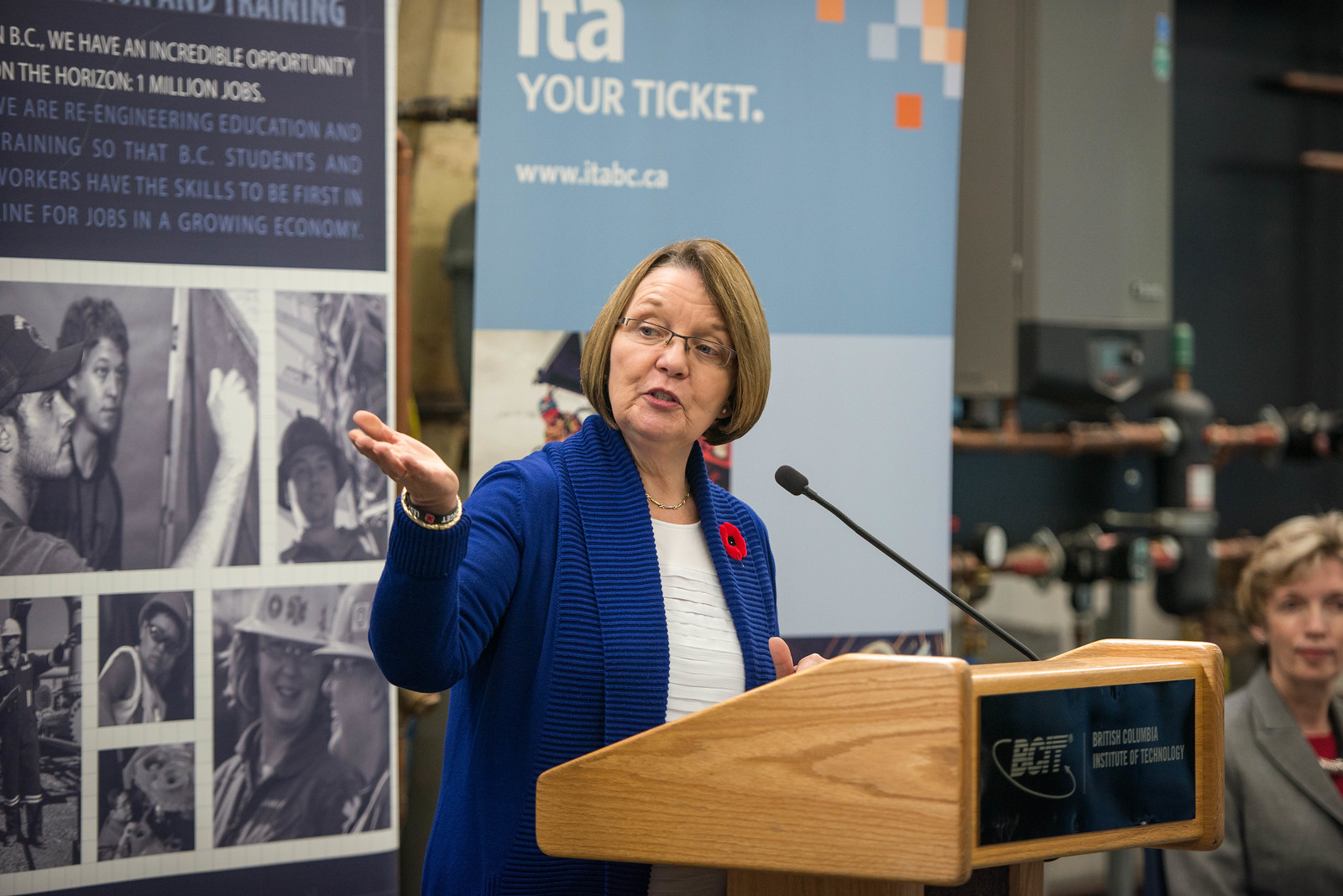The image features a middle-aged woman standing at a podium that prominently displays "BCIT" on the front, signifying the British Columbia Institute of Technology. She appears to be speaking, evidenced by her slightly open mouth and attentive posture. The woman is dressed in a dark blue suit jacket adorned with a red poppy flower pin on her left lapel, a white blouse, and a stylish necklace. She has short to medium brown hair styled in a bob, wears glasses, and a watch on her right wrist. Her body is angled to the right of the image, but she turns her head to the left, engaging with the audience to her right, while her right hand is lifted, arm bent, with her hand flat, adding emphasis to her speech.

Behind her are several banners and displays. One banner reads, "In BC, we have an incredible opportunity" and "One million jobs." Another emphasizes the theme of re-engineering education, stating, "We are re-engineering education and training so that BC students and workers have the skills to be first in line for jobs in a growing economy." Some displays feature black and white photographs of workers in hard hats, suggesting an industrial or technical educational focus. In the background, under soft lighting, another woman is visible, sitting and dressed in a gray suit jacket with short blonde hair, behind whom mechanical elements like pipes, valves, and tanks can be seen, enhancing the technical and professional ambiance of the scene.